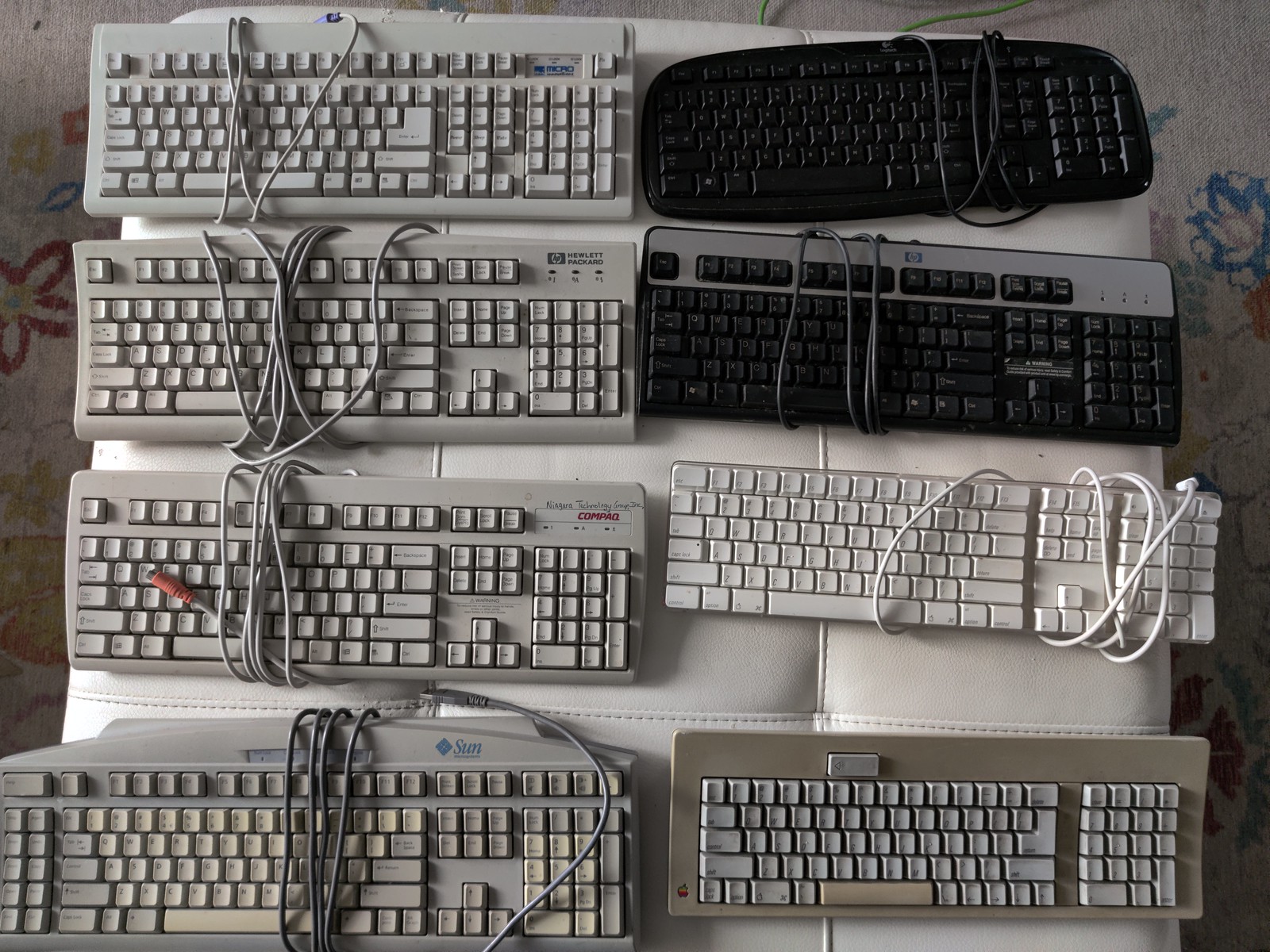The color photograph, rendered in a nearly black and white scheme with hints of sepia and greyish-brown tones, depicts eight keyboards arranged in two stacks of four on a quilted, leather-like, cream-colored surface. The stack to the left consists predominantly of keyboards in grey tones, while the stack on the right features keyboards of varying colors — the top two being black, the third a lighter grey, and the bottom one a beige with greyish-white keys.

Each keyboard varies in size, shape, and brand identification. Within the details, several cords are visible, wrapped around most keyboards except the bottom right. Notable keyboards include a cream-colored one at the bottom right with a red and white Apple logo at the bottom left corner, and a black keyboard at the top right displaying a blue HP logo with a silver rim. The grey keyboard on the left stack bears the Compaq logo in red on its top right, while the grey one directly at the bottom left features the Sun logo in blue.

The leather-like surface rests atop a grey background that features a floral pattern, distinguished by large red, blue, and yellow splotches resembling petals, particularly prominent on the left side, with additional blue markings scattered on the right and pale green lines near the top, adding a touch of color to the subdued palette.